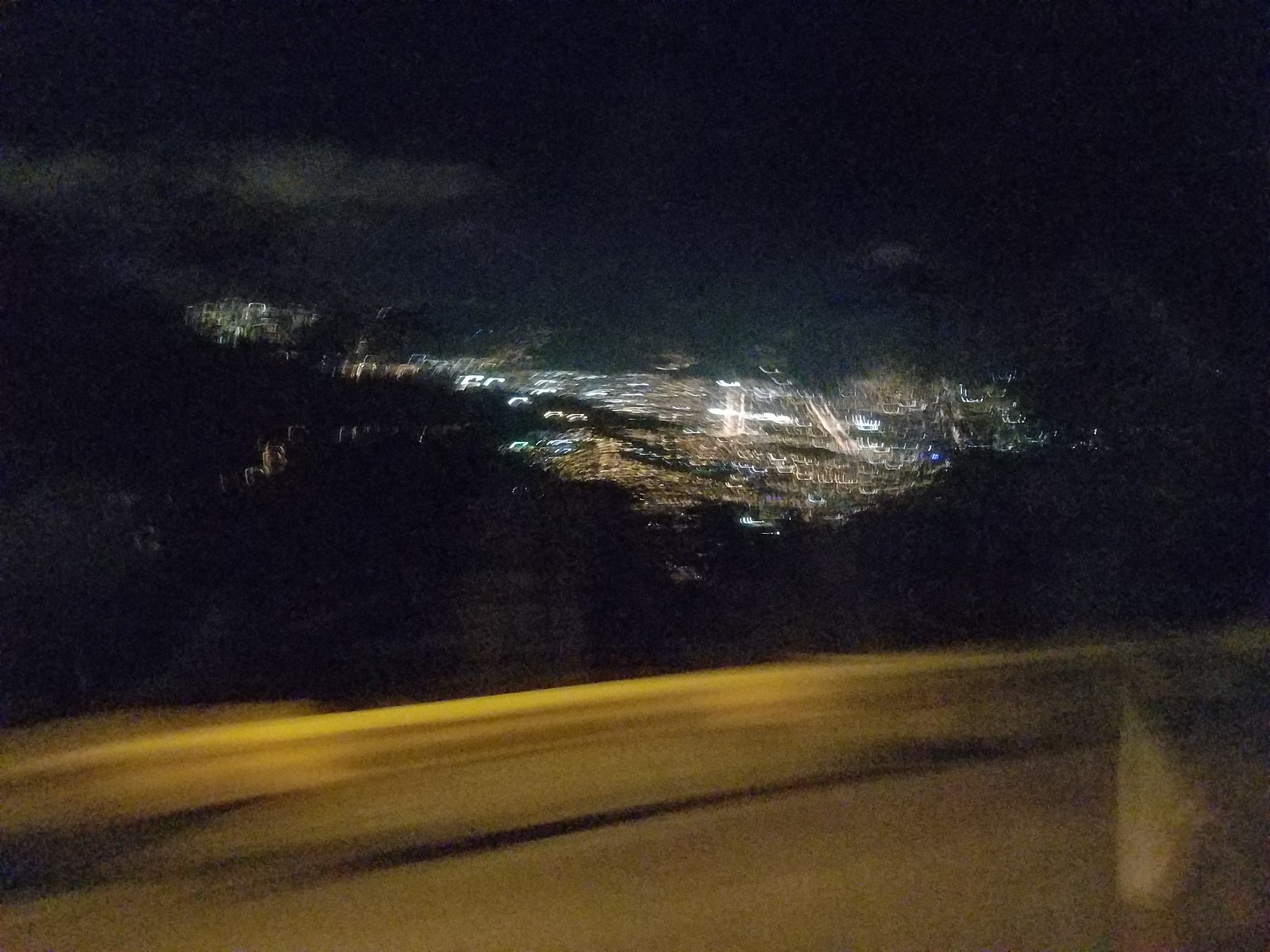A photograph showcasing a night-time cityscape from a higher elevation, captured from within a moving vehicle, resulting in a slight motion blur. The twinkling city lights create a vibrant, blurry mosaic, while the white and yellow lights at the bottom of the image delineate the road below. A glass reflection in the bottom right corner adds depth, further indicating this photo was taken behind a window. Silhouettes of trees frame the luminous city in the distance, enhancing the composition with a touch of nature amidst the urban sprawl.